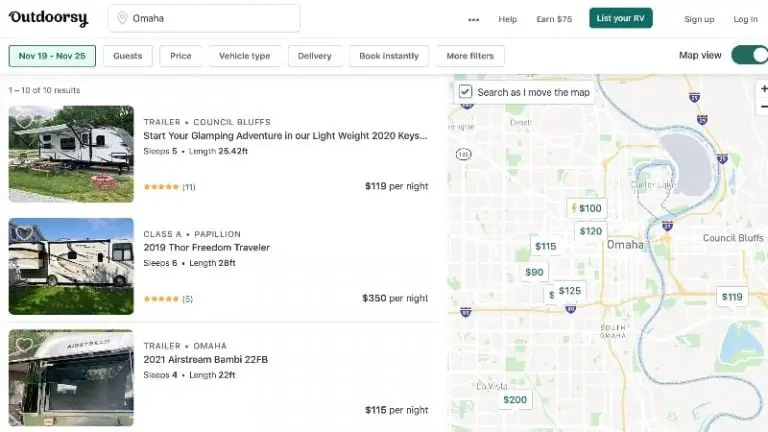This image is a screenshot of a laptop displaying the Outdoorsy application, primarily designed on a white background. Outdoorsy is a platform for renting RVs and trailers. In the upper-right corner of the interface, there are several interactive buttons labeled 'Help,' 'List Your RV,' 'Sign Up,' and 'Log In.' Beneath these options, users can find search buttons to refine their inquiry on available RVs and trailers. The main section displays various listings, each accompanied by a photograph. For example, one listing features a trailer available for rent at $119 per night. Adjacent to this listing, a map highlights the locations where these RVs and trailers are available for rent.